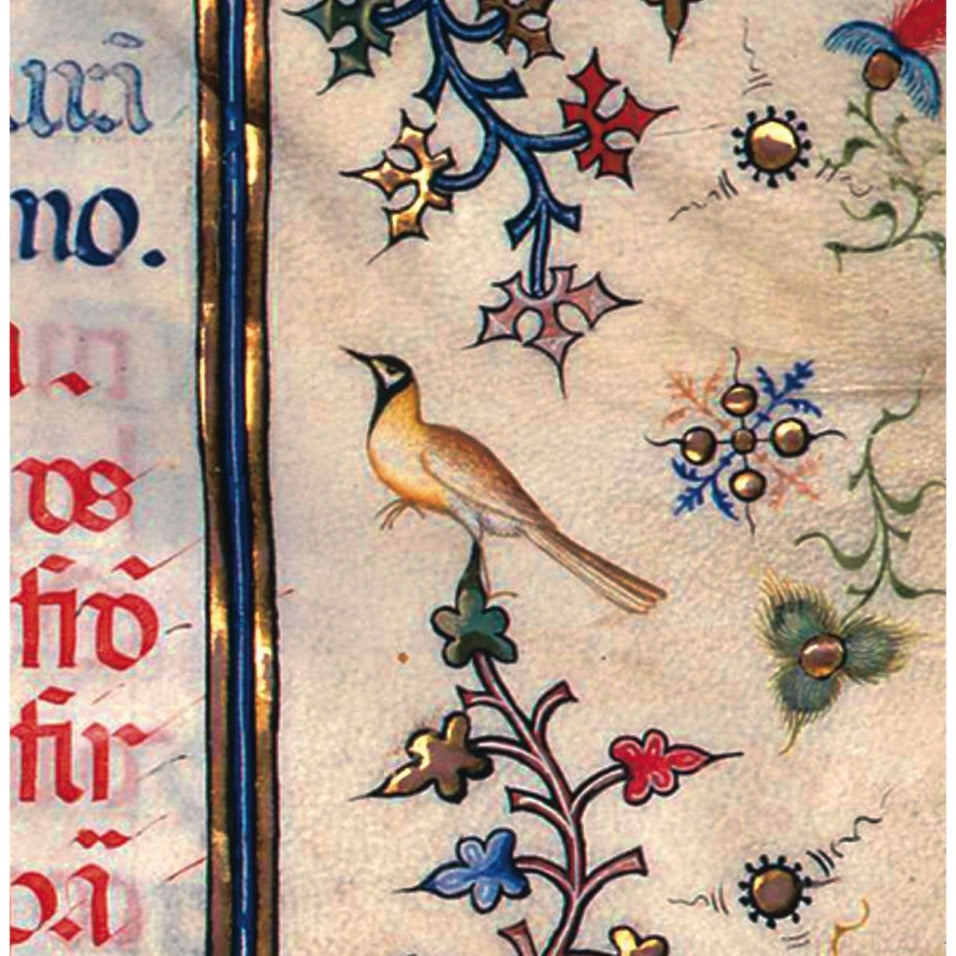This detailed close-up image appears to be from an old, medieval illustrated book or atlas, with an ornate illustration dominating the scene. The right side of the page features a golden bird with a black head and white markings, perched atop an intricate, abstracted stem adorned with leaves in various colors, including blue, red, gold, and green. Surrounding it are additional leaves and shapes that resemble biological organisms. The left side of the image is filled with an intricate calligraphic text, partially visible and featuring lines in blue and red ink. A vertical stripe with a pattern of gold and blue runs parallel to the text. The overall impression is of a meticulously hand-painted, richly colored illustration typical of ancient manuscripts, presenting a fascinating blend of flora and fauna in vibrant hues against a backdrop of elegant script.